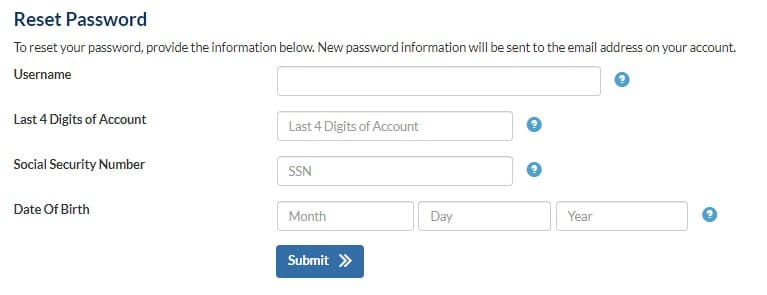The image depicts a "Reset Password" screen, prominently titled at the top left with each word capitalized. Beneath this title, there is a guiding message: "To reset your password, provide the information below. New password information will be sent to the email address on your account."

The form consists of several fields where users need to input their details:

1. **Username**: A labeled box to enter your username.
2. **Last Four Digits of the Account**: A box requesting the last four digits of your account number.
3. **Social Security Number (SSN)**: A designated box for your Social Security Number.
4. **Date of Birth**: Separate boxes to input the month, day, and year of your birth.

Adjacent to each field is a small blue circle with a question mark, providing additional help or explanations if needed. This can be useful for clarifying terms like "last four digits of the account" or "SSN."

At the bottom of the screen, there is a blue "Submit" button with white text, intended to finalize the process after all required information is entered.